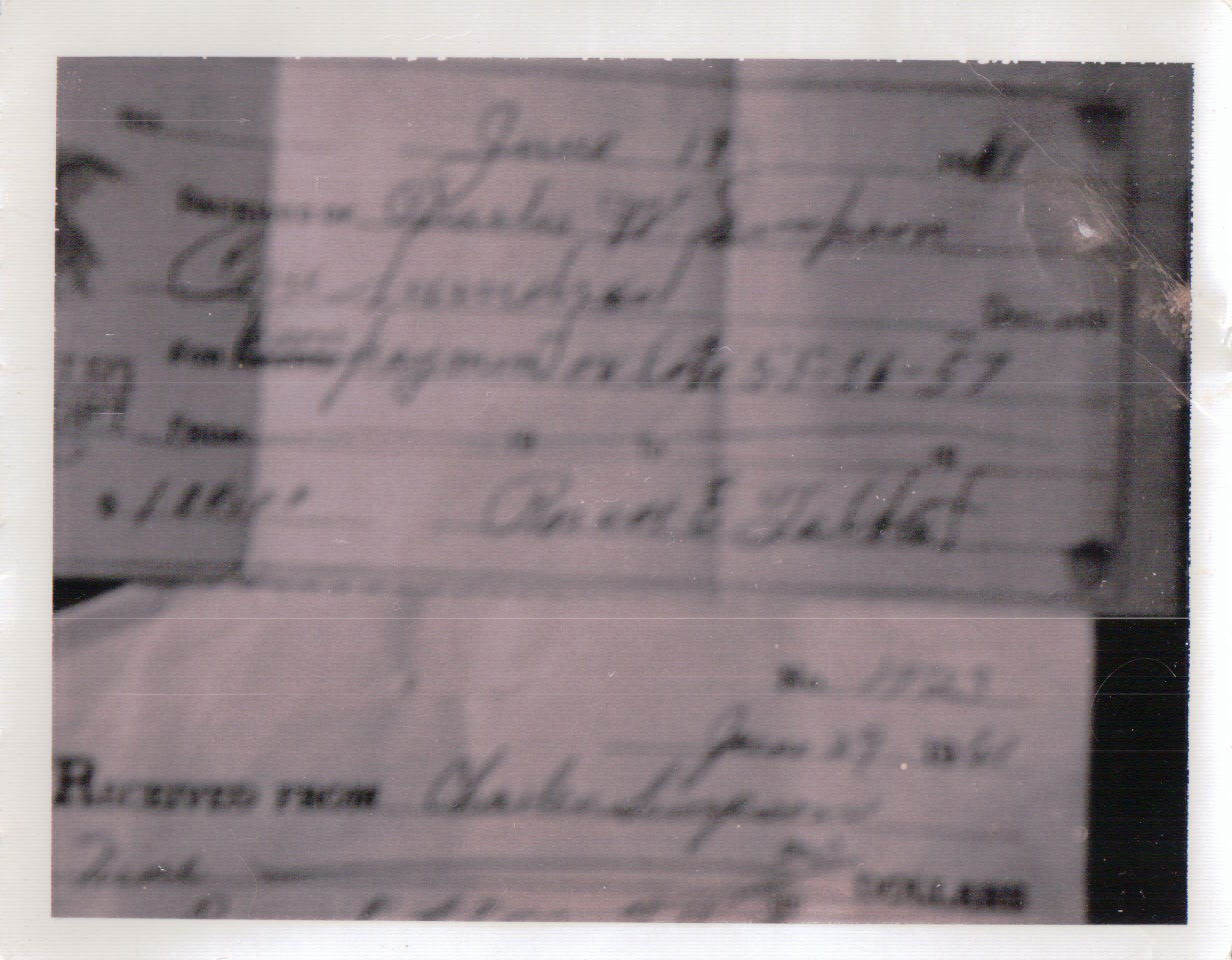This is a very blurry, out-of-focus photograph bordered by white, reminiscent of a Polaroid picture. In the upper right corner, there appears to be a small scuff or scratch on the photo. The image displays two large sheets of paper, which look like old-fashioned checks, one placed above the other. Both checks are adorned with lots of cursive writing that is mostly illegible due to the blurriness. However, each check appears to have a date written on it, and the bottom check has a legible phrase "received from." Despite the unclear details, the checks give off a vintage feel.